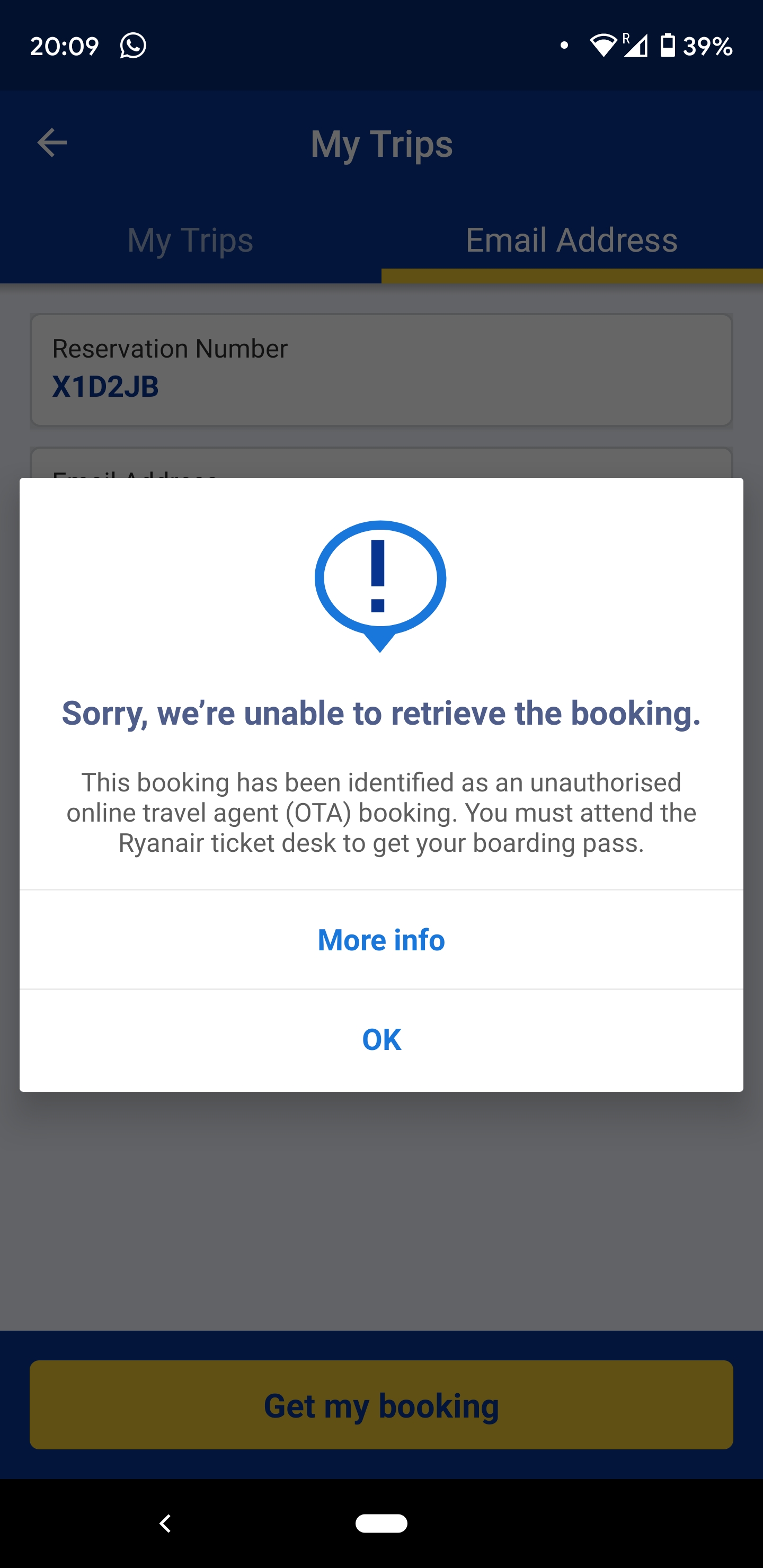The image is a screenshot from a cell phone, with the top left corner displaying the time as 20:09 alongside a small white icon of a telephone. To the right, the battery indicator shows a 39% charge with a white battery icon. The background is slightly blurred and dark, featuring a blue gradient at the top with the words "My Trips" in white text displayed twice, once on the left and once more prominently on the right.

Below this, an email address is highlighted in yellow. Further down, the text reads "Reservation Number X1D2JB," followed by a white box containing a circle with an exclamation mark inside it. Beneath this, the text says, "Sorry, we're unable to retrieve the booking. This booking has been identified as an unauthorized online travel agent (OTA) booking. You must attend the RYANAIR ticket desk to get your boarding pass."

At the bottom of the image, additional clickable options include "More info" and "OK," both in blue text, as well as a yellow button labeled "Get My Booking."